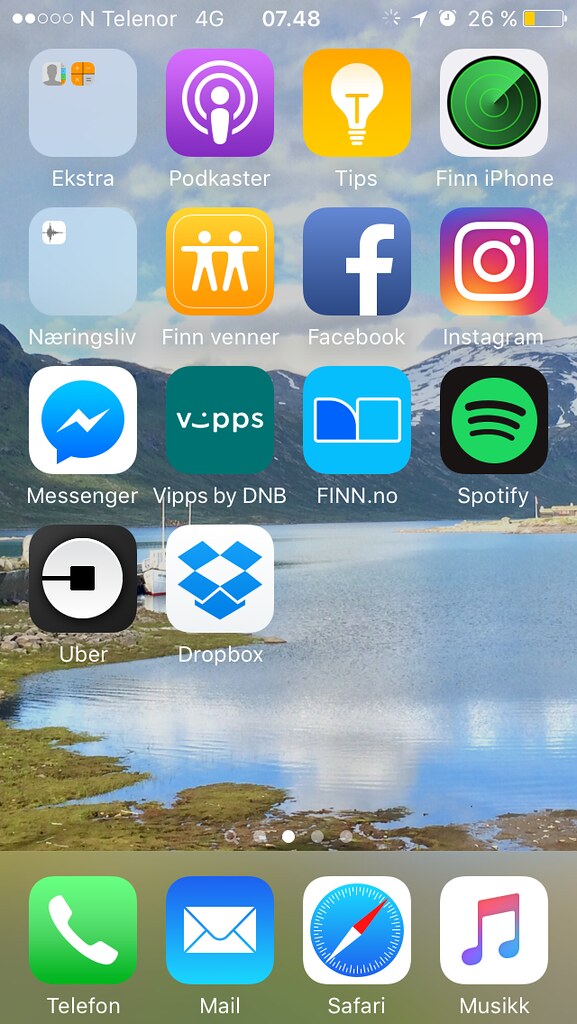The image features a home screen, likely from an iPhone, decked with various application icons overlaid on a stunning scenic background. The background showcases a picturesque view with a serene blue lake bordered by lush green grassy banks. In the distance, rugged snow-capped mountains rise majestically against the horizon, adding to the image's natural beauty.

At the top of the screen, the status bar displays the network provider as N-Telenor 4G. The time reads 7:48, and the battery indicator shows a 26% charge, confirming that this is indeed a mobile phone.

The home screen is populated with an array of app icons. Prominently featured is the "FiniPhone" app, suggesting the device's identity as an iPhone. Beside it, there's an icon of a light bulb labeled "Tips," followed by a podcast app, and another icon simply named "Extra." The app array also includes popular social and utility apps like FinVeneer, Facebook, Instagram, Spotify, Dropbox, Uber, Messenger, and Nehring Sliv. Financial and service apps such as Vips by DNB and Fin.no are also visible.

At the bottom of the screen, the dock contains four essential app icons: a green telephone symbol for calls, an email icon labeled "Mail," the Safari browser, and a music app.